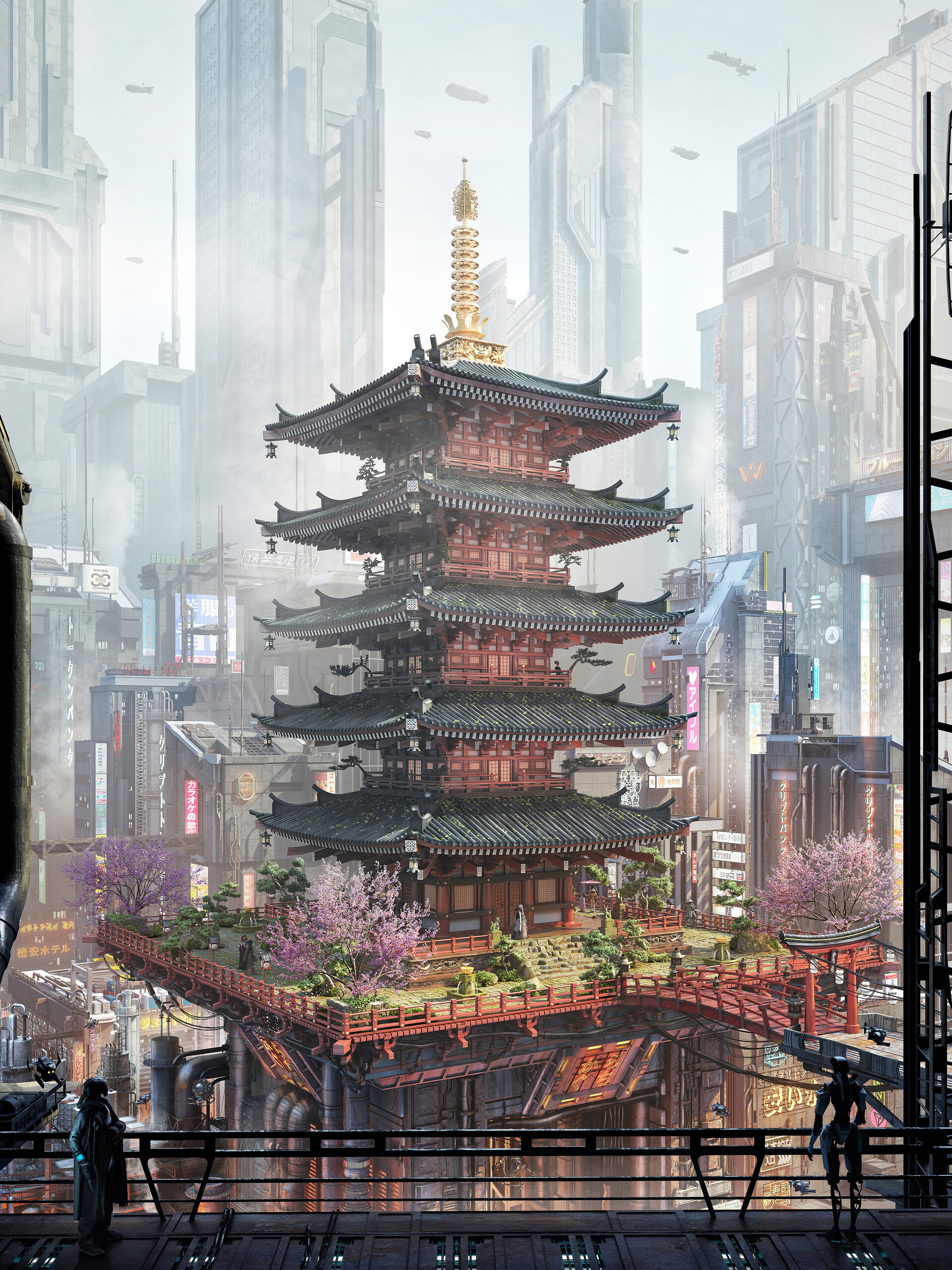This captivating, digitally or AI-generated color portrait depicts an intricate structure at its center, featuring five stacked pagoda-style roofs. Each tier is interspersed with brown segments adorned with windows, doors, and balconies. The middle section of the building showcases a large balcony lush with trees and plants, creating a vibrant focal point. Crowning the structure is a striking gold spire, adding a touch of elegance. In the background, several tall buildings with a faded, washed-out appearance rise into the sky, some adorned with vertical signs inscribed in an Asian alphabet. A black metal fence runs along the foreground, where two silhouetted figures stand. The figure on the right, with a distinctively robotic appearance, contrasts sharply with its companion, further enhancing the image's surreal and otherworldly ambiance.